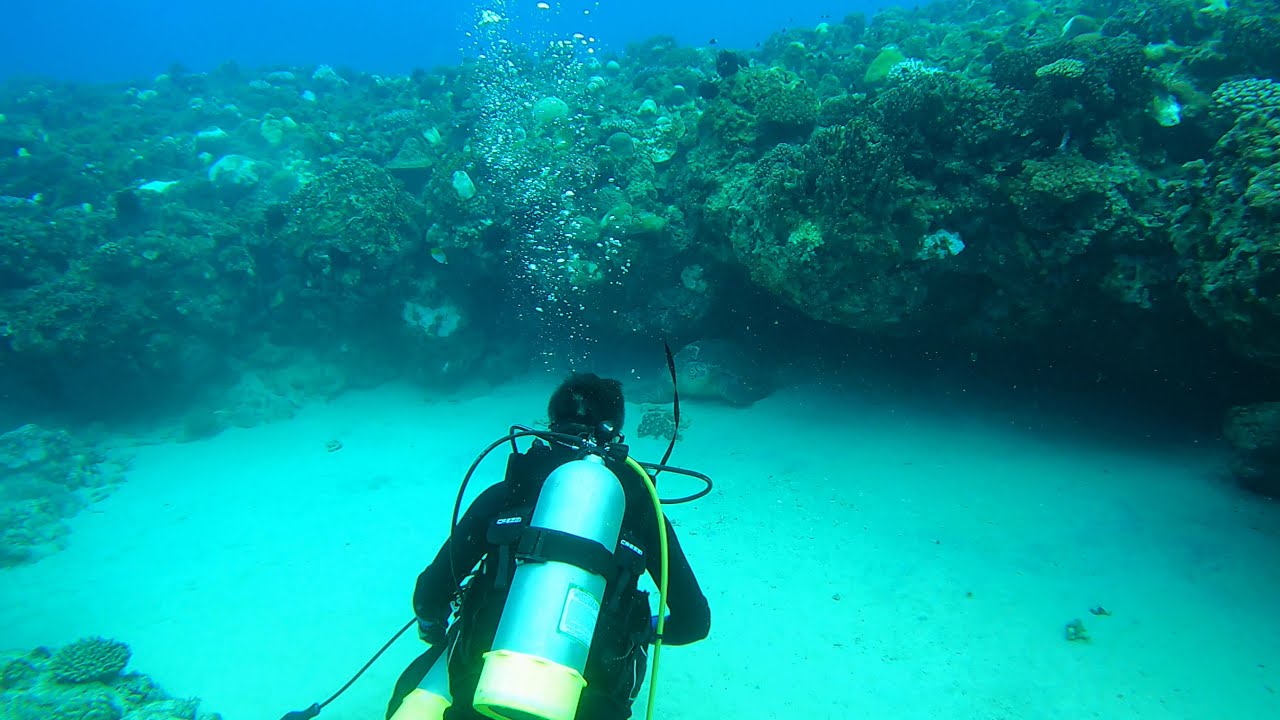In this rectangular underwater photograph, a diver is captured in the center of the image, fully immersed in an aquamarine oceanic environment that transitions to a darker blue towards the top. The diver, clad in black, has a blue and yellow oxygen cylinder strapped to his back, from which various tubes—yellow, green, and black—are emanating, ensuring his air supply. Numerous air bubbles are visible, originating from the diver's helmet or mouth area, rising towards the surface. The seafloor, appearing in shades of light blue, features a prominent coral reef directly in front of the diver, displaying dark green hues and adorned with various ocean plants and rocks. Additional coral extends to the left-hand bottom side of the photo, framing the serene underwater landscape devoid of any visible fish or other marine life.